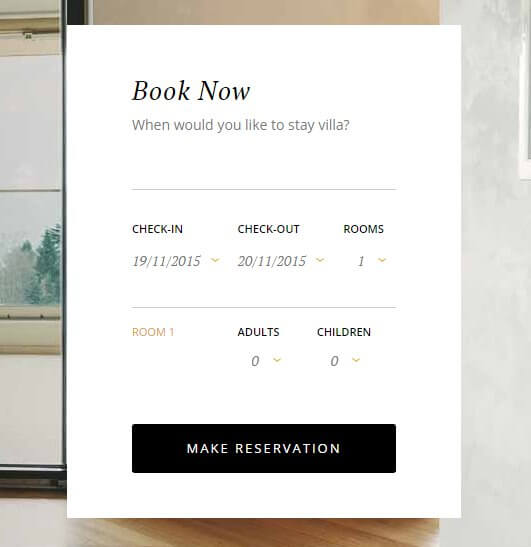The image displays a reservation interface for a villa booking. Visible details include an option to "Book Now" with fields prompting "When would you like to stay?". The check-in date is set to November 19th, 2015, and the check-out date is November 20th, 2015. The reservation request is for one room, accommodating zero adults and zero children. The colors present in the interface include white, black, brown, and grey, contributing to a clean and sophisticated design. Additionally, there is a window pane situated on the left side of the image, adding to the overall aesthetic with natural light.